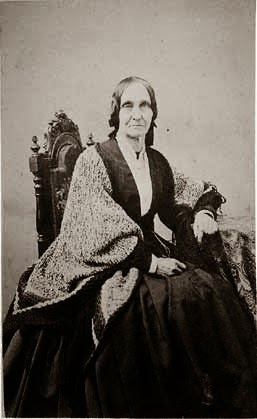This black-and-white photograph captures an elderly woman sitting on an antique, dark-colored chair against a gray wall. She appears to be looking directly at the photographer with a neutral to unhappy expression. Her attire includes a dark vest-like dress that reaches down widely, complemented by a light-colored sweater with a black hem. Her right arm rests on the chair's armrest while her left hand is placed on her lap. The chair has an old-fashioned design, featuring two distinct points on the sides and one in the middle. The woman's hair is short, likely brown, and falls to her shoulders. The overall composition of the photo suggests an antique and somber atmosphere.